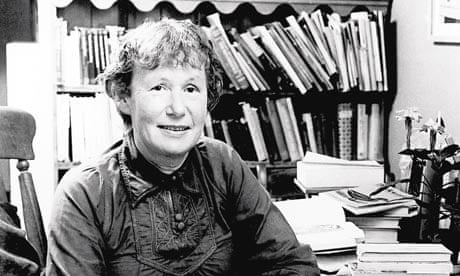The black and white hyper-realistic photograph captures a middle-aged woman, likely in her 50s, seated slightly off-center at a desk within a study. Her short, unkempt, bushy hair frames her face as she gazes directly at the camera with a gentle smile. She wears an older-style button-up collared shirt with long sleeves, possibly adorned with some decorations around the collar. The desk in front of her is cluttered with open textbooks and hardback books, all in a state of disarray. A partially visible wooden chair, presumably the one she is seated on, can be seen to her left. Behind her, the bookshelf appears almost overflowing with an eclectic and somewhat haphazard collection of books. To the right of her desk, amidst the scattered books, there is an indistinct object that might be a small plant or flowers, barely discernible in the monochromatic palette of the photograph.